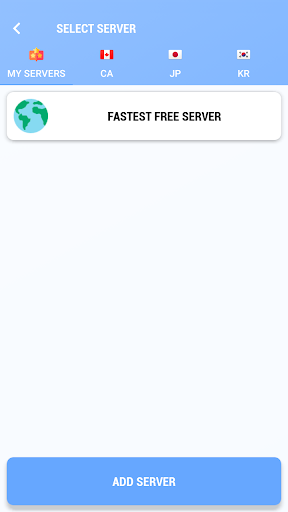At the very top of the image, the background features a light blue, elongated rectangle. Within this rectangle, there is a small arrow pointing to the left, accompanied by the text "Select Server." 

Below this section, there is a small orange and yellow box with the white text "My Servers" written beneath it. 

To the right of this, there is an image of the Canadian flag, characterized by its distinct red and white stripes and a prominent red maple leaf in the center. Positioned directly below the flag are the letters "CA" indicating Canada.

Next to the Canadian flag is the Japanese flag, which consists of a white background with a central red circle. Below this flag are the initials "JP" for Japan.

To the right of the Japanese flag, there is a white square containing five black dots, with the center dot being the largest. The text "KR" is displayed underneath, representing South Korea.

Following this, there is a square depicting an image of Earth, showcasing blue water and green landmasses. Adjacent to this image are the words "FASTEST FREE SERVER" in uppercase black letters.

Finally, at the bottom of the image, there is a blue rectangle with the uppercase white text "ADD SERVER" inside.